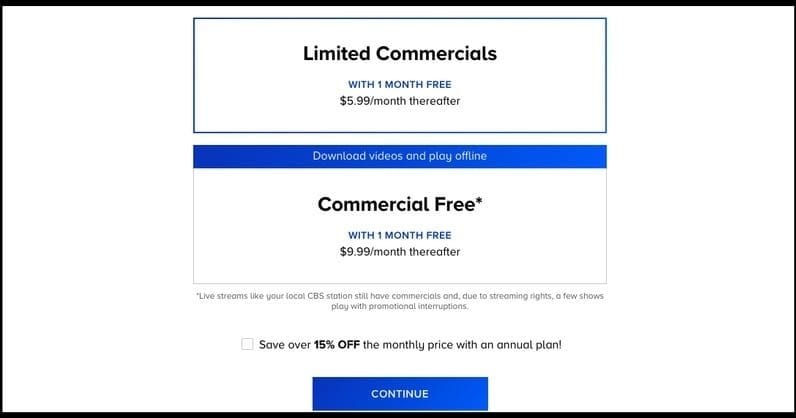This image is a screenshot from a streaming service, featuring a large white rectangular interface bordered in black. In the central part of the screenshot, there are two prominent rectangular sections, one positioned above the other.

The top rectangle is highlighted with a blue outline and contains bold black text stating "Limited Commercials." Below this title, in blue capital letters, it reads "WITH ONE MONTH FREE." Further down, smaller black text indicates the pricing, "$5.99 per month thereafter."

The second rectangle, positioned below the first, features a blue bar at the top, containing text that reads "Download Videos and Play Offline." Directly underneath, the text states "Commercial Free" followed by an asterisk. It continues with the offer "WITH ONE MONTH FREE" and the price "$9.99 per month thereafter."

Beneath these two main sections, additional explanatory text clarifies, "Live streams like your local CBS station still have commercials, and due to streaming rights, a few shows play with promotional interruptions."

At the bottom of the screenshot, there is a blue button labeled "CONTINUE."